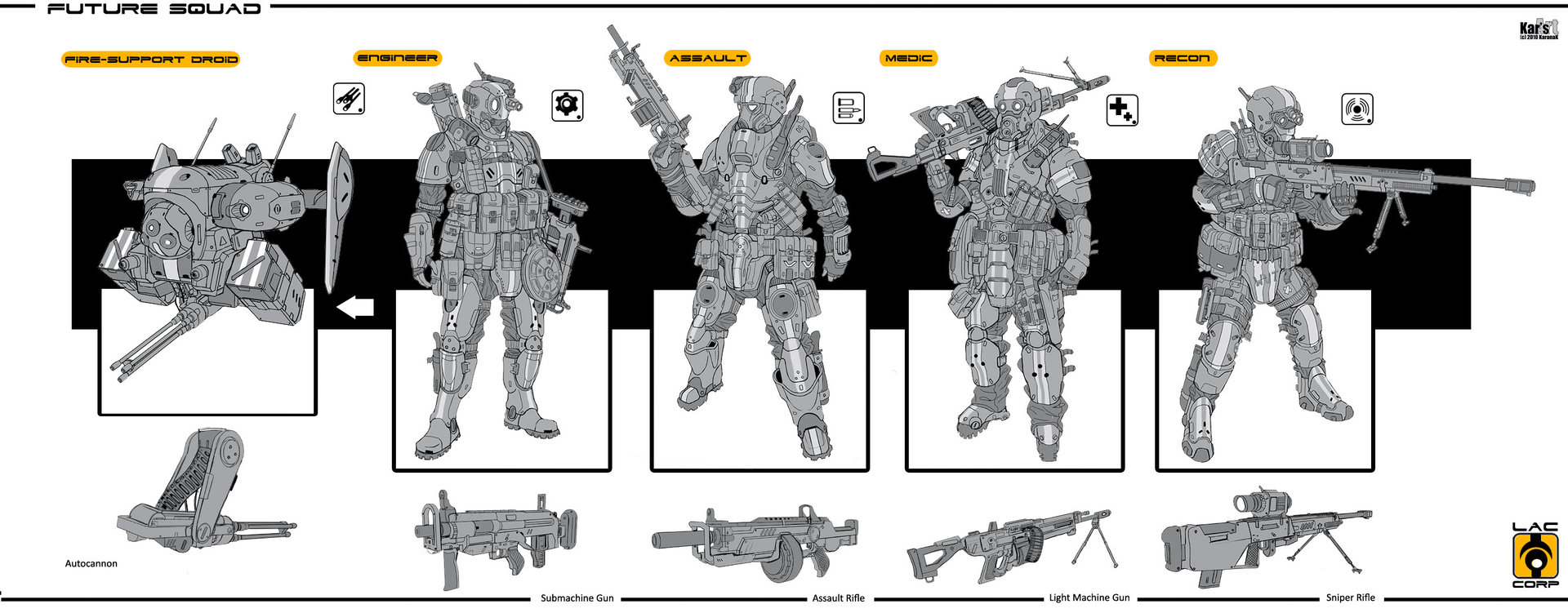The image is a detailed, monochromatic sketch in black ink with gray and white shading, depicting futuristic character designs labeled "Future Squad." The characters, appearing on what looks like a character selection screen from a video game, include both humanoid figures and a robot. The first figure is identified as a "Fire Support Droid," showcasing a heavily armored, non-human robot. Following this are four humanoid characters completely covered in high-tech, metallic armor, reminiscent of Iron Man suits, with no visible faces or exposed skin. These figures are labeled according to their roles: "Engineer," "Assault," "Medic," and "Recon," each with distinct weaponry corresponding to their role. Below these characters, additional close-up illustrations of various guns are displayed, labeled as sub-machine guns, assault rifles, light machine guns, and sniper rifles. The scene is filled with various symbols and logos, including one for "LAC Corp" in black and gold, and another partially legible logo in the top right corner. The overall impression is of a highly detailed, futuristic military squad, equipped with advanced weaponry and gear.